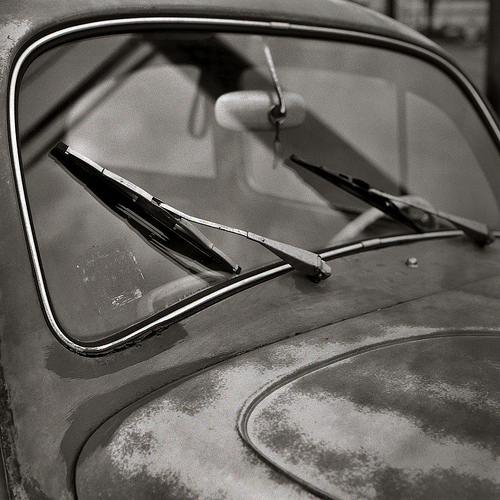This detailed black and white photograph captures the front of a vintage car, possibly a 1950s VW Beetle, showcasing its aged charm and need for restoration. The windshield, which curves gracefully at the edges, is primarily clear but features remnants of a sticker in the lower left corner. Two windshield wipers are positioned to the left, and a rear-view mirror hangs behind the glass. The hood exhibits significant wear, with patches of rust and the underlying metal exposed where the dark paint has eroded or been sanded down. The overall tone of the car is dark, with areas that appear silvery or white due to the patina. In the background, a blurry mix of gray and black adds depth to the image.